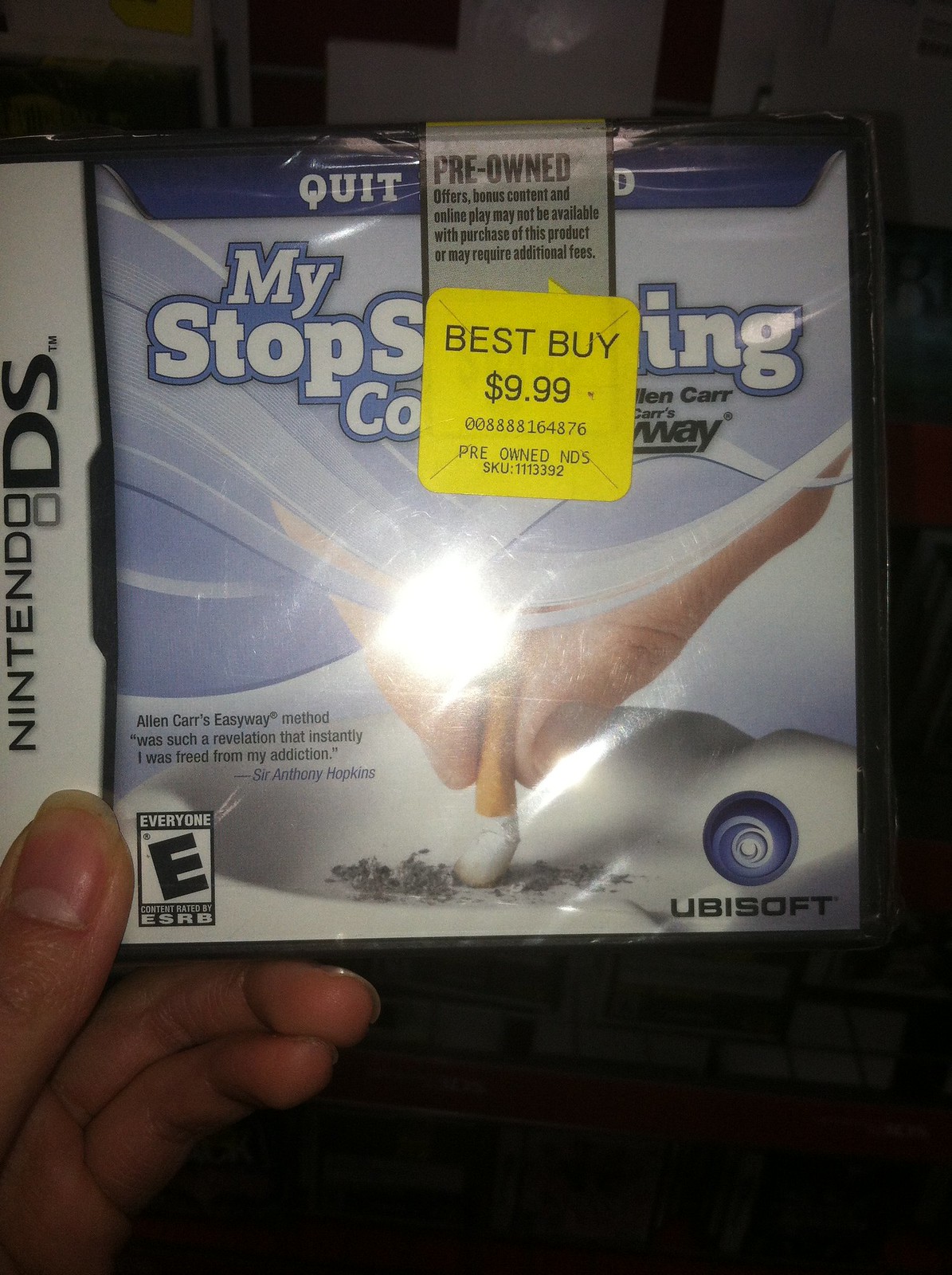This photograph features a Nintendo DS game case being held by a person with fair skin and unpolished fingernails, visible in the lower left-hand corner of the image. The game, a pre-owned item from Best Buy priced at $9.99, is encased in plastic packaging with two stickers at the top center partially obscuring the title. The first sticker, in black text, states "pre-owned, offers bonus content, and online play may not be available with purchase of this product or may require additional fees." Below it is a yellow sticker displaying "Best Buy, $9.99, 00888164876, pre-owned NDS," along with a SKU. Despite the stickers, one can make out that the game is titled "My Stop Smoking Coach," based on the visible text. The cover image features gray swoops and a hand stubbing out a cigarette, indicating its purpose as a quit-smoking aid. Additional details include an E for Everyone rating in the bottom left corner and the Ubisoft logo in the bottom right. The phrase "Alan Carr's easy way method was such a revelation that instantly I was freed from my addiction, Sir Anthony Hopkins" suggests a testimonial for the effectiveness of the method depicted in the game.